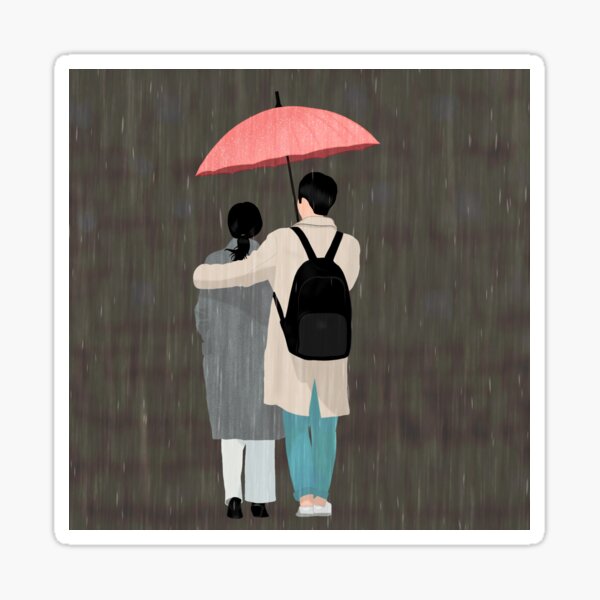This detailed painting depicts two people under a vibrant red umbrella in the rain. The rain drizzles down the entire image, creating white streaks against a solid gray background. The scene is framed by a white square border with rounded edges. 

The pair, a possible man and woman, are viewed from behind, adding to the sense of anonymity. The woman, identifiable by her long black hair tied in a ponytail, wears a gray coat—perhaps a fur coat—paired with white pants and black shoes. The man beside her has short black hair and light skin, and dons a tan coat with a black backpack that has a gray pocket. He also wears blue pants and white shoes. 

The man's protective arm wraps around the woman as he holds up the umbrella, its black handle and red covering contrasting sharply with the muted tones of their clothing and the background. The couple is set against a gray backdrop where colors mix with the rain, blending blue, purple, and green hues, although no distinct details can be made out. The bright red umbrella and the man's blue pants stand out vividly amidst the otherwise subdued palette, adding a striking contrast to the rainy scene.